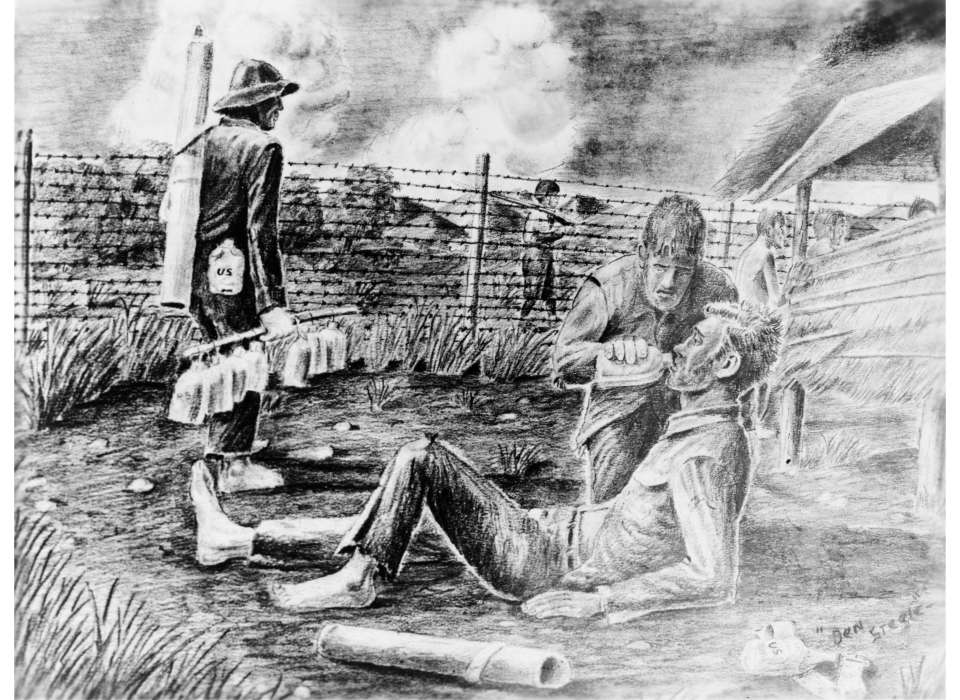This detailed graphite or charcoal illustration depicts a somber military scene, possibly a war camp, set against a backdrop of dark clouds and a barbed wire fence. Beyond the fence, a couple of figures are faintly visible, including a young male holding a rifle over his shoulder, suggesting a tense environment. 

In the foreground, the primary focus is on three men, each conveying a sense of hardship and struggle. To the left, one man, dressed in a military uniform with a hat, is walking away and facing the fence. He has a strap over one shoulder, carrying a long rod with several canteens of water. His attire includes a long sleeve shirt and pants, and he looks like he might be barefoot.

Central to the composition is a poignant interaction between two men. One man, appearing sick or injured, lies on the ground without shoes or socks, his pants ripped at the ends. He is partially sitting up to drink from a canteen held by another man kneeling beside him. Both men have concerned, weary expressions, emphasizing their middle-aged appearance and the gravity of the situation.

This detailed and evocative scene captures the raw emotion and bleak reality of wartime circumstances, highlighting moments of compassion amidst the chaos.